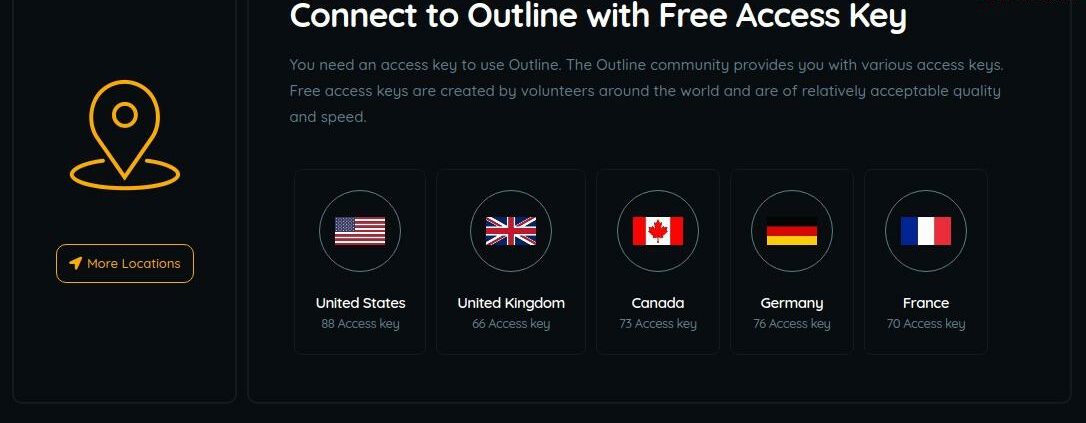The image features a black rectangular box that is oriented more horizontally than vertically. The text within the box is in white and reads, "Connect to Outline with free access key." Below this text, there is a peculiar icon resembling a map pin, which is black with gold outlines, featuring a gold circle and a gold plate near its point. In small text at the point of the pin, it says, "More locations." 

Beneath the icon and text, there is an actionable section indicating that "You need an access key to use Outline," and mentions that "the online community provides you with various access keys." Further details are available in explanatory text below this section.

At the bottom of the image, five flags are displayed in a row, each representing a different country: the United States, the United Kingdom, Canada, Germany, and France. Under each flag, the number of available access keys is listed: 88 for the United States, 56 for the United Kingdom, 73 for Canada, 76 for Germany, and 70 for France. An additional note encourages users to check other locations on the left side if their country is not listed.